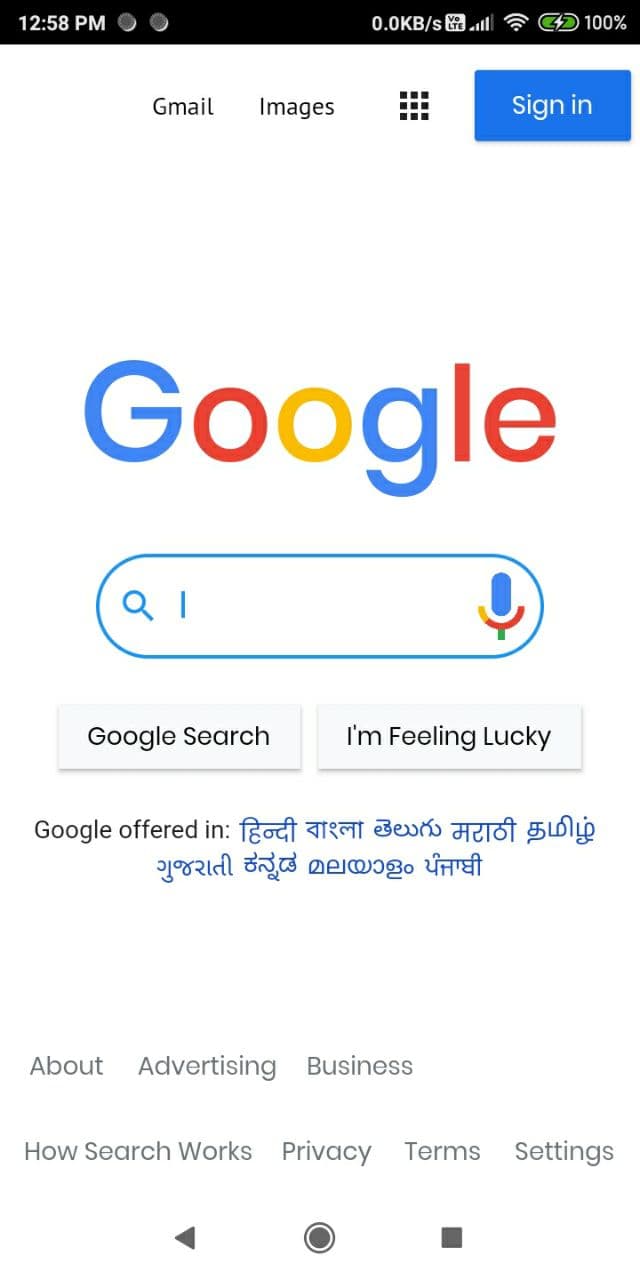This image captures a screenshot from a cell phone, evident by the visible status bar at the top showing the time as 12:58 PM and the battery at a full 100% charge. At the very top of the screen, the word "Gmail" is displayed prominently, followed by the "Images" tab, and an icon consisting of multi-square tiles forming a larger square. Next to this section is a blue "Sign in" button.

Beneath this section, there's a white space that features the Google logo, which is displayed in its customary multicolored letters. However, an unusual detail is that the letters are slightly altered: the capital 'G' is blue, the first 'o' is red, the second 'o' is yellow, the 'g' is blue, but both the 'L' and 'e' are red instead of the 'L' being green as normally seen.

Below the Google logo is the search bar, which includes a microphone icon on the right end for voice searches. Two buttons are positioned underneath the search bar: "Google Search" and "I'm Feeling Lucky." Lower on the screen, there are quick links for About, Advertising, and Business information.